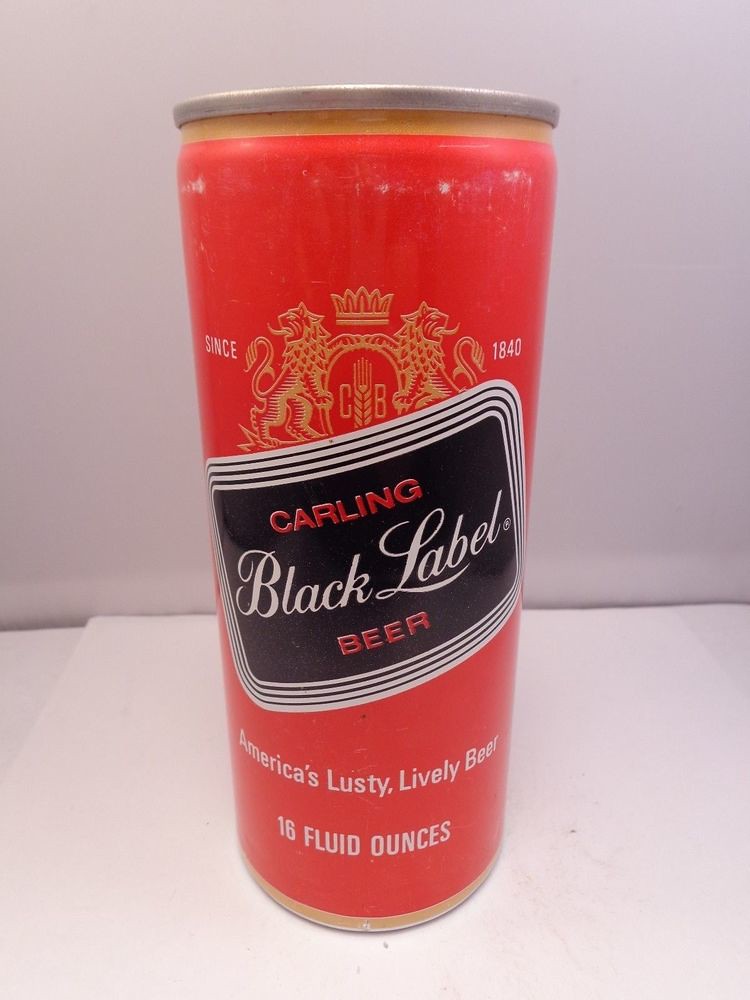This is a detailed, color, close-up photograph taken indoors of a Carling Beer can positioned on a white table against a white wall. The can is fully in the frame, showcasing its front label. The can features a silver metallic top, below which is a thin mustard-yellow stripe separating the top from the main body of the can. The main body sports a vibrant orangey-red color which wraps around the entire background. 

Dominating the upper part of the can is a coat of arms that includes two lions standing on either side of a central crest, their tongues out and tails curling back towards their bodies. The lions face each other, standing upright with their paws on the crest. The crest displays a crown with five triangular points and includes a circle featuring four rods and a heart, linked by diagonal rectangles. Beneath this emblem, it is inscribed with "Since 1840" in white text.

Immediately below the coat of arms, in the middle section, there is a bold black rectangular label with multiple alternating thin white and black stripes bordering it. This label displays the word "Carling" in stark white text, followed by "Black Label" written in white stylized, italicized cursive, and finally "Beer" in red text beneath it. 

Towards the bottom of the can, under the label, white text declares, "America's Lusty, Lively Beer," alongside the volume size of "16 fluid ounces." The base of the can is again circled by a thin mustard-yellow stripe, adding another layer of detail to its design.